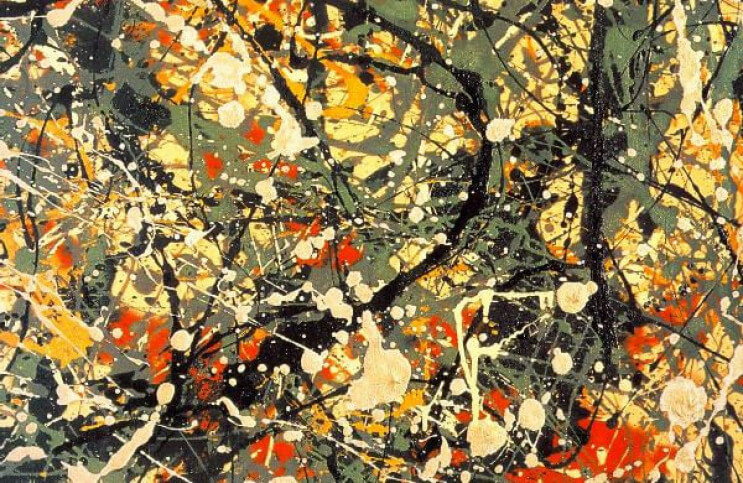This is an abstract painting characterized by an array of dynamic splashes and splatters of paint. Dominated by a chaotic but intriguing mix of colors, the artwork features pronounced black streaks that cascade down the middle, accompanied by vibrant splatters of red, yellow, and orange. Interwoven into the composition are subtle touches of green and dark green, mingling with areas of dark gray and creamy white. The overall impression is somewhat vine-like, with the diverse colors and textures merging and diverging across a grayish background. The painting emanates energy and spontaneity, capturing a sense of wild, unrestrained creativity.